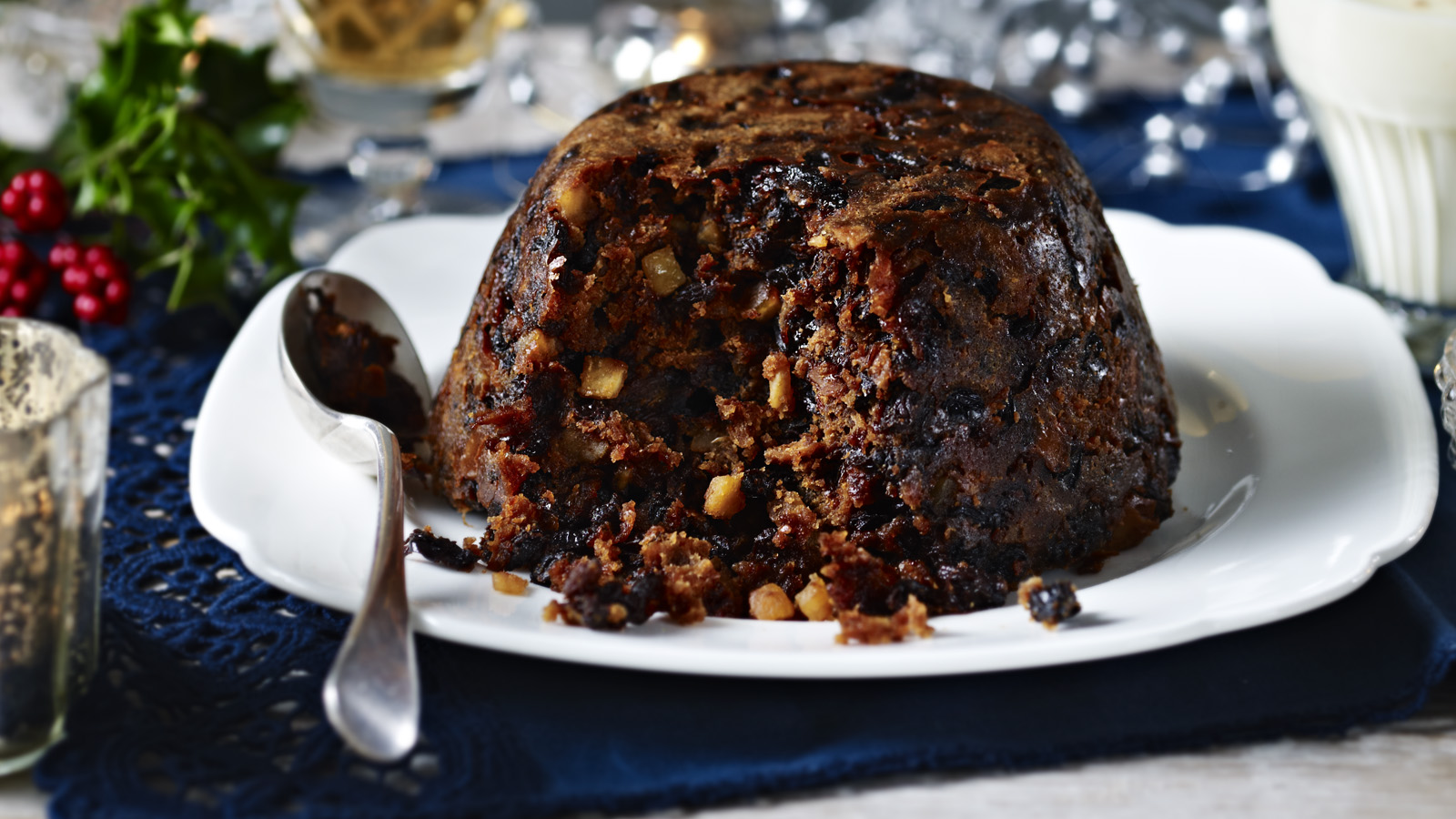The photograph depicts a dessert setting, centered around a brown, dome-shaped cake that sits on a white porcelain plate. A large scoop has been taken from the front-left side of the cake, revealing a textured interior with bits of raisins and possibly chopped nuts, which are light tan or yellowish in color. The plate is accompanied by a silver spoon resting on its left side. This setup is presented on a knitted blue lacy placemat or tablecloth. Surrounding the main focus, there are red berries with green leaves visible in the background, along with various indistinct glass and silverware items, contributing to a formal dinner setting ambiance.